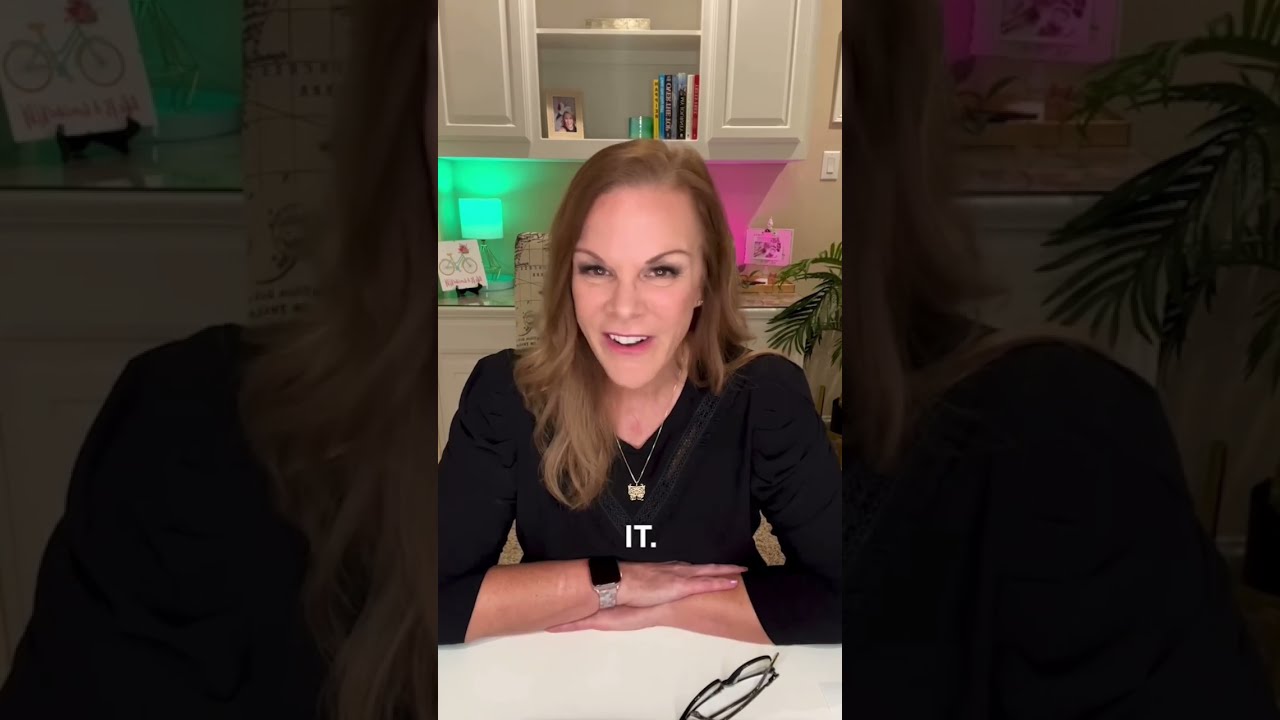In this image, you see a Caucasian woman with light brown, slightly wavy hair that curls at the bottom, seated at a bright white table. She is wearing a black, long-sleeved top with the word "IT" visible in the middle, and a smart watch on her right wrist. Her arms are crossed on the table in front of her, where a pair of black, folded reading glasses are also placed. She has a thin face accentuated by heavy eye makeup and is adorned with a necklace featuring a butterfly pendant. The woman is looking directly at the camera with her mouth slightly open as if in mid-conversation, revealing her top front teeth. Behind her, the setting resembles a kitchen or office space with white cabinets, a stone countertop, and various items including books on white shelving. The background is lit with contrasting green and pink lights.